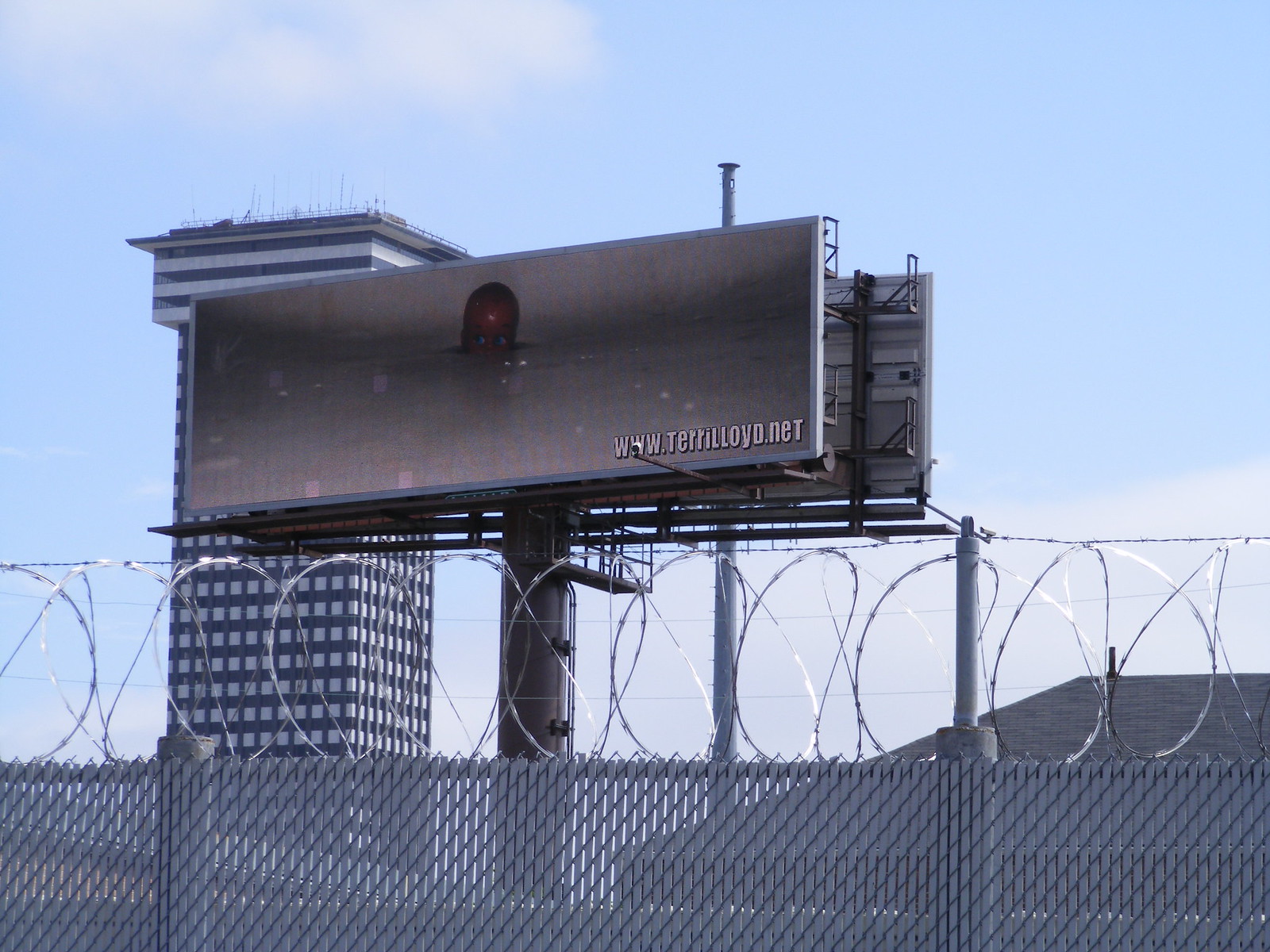The photograph captures an outdoor scene featuring a foreground dominated by a chain-link fence topped with tightly coiled, sharp barbed wire. Rising behind the fence is a tall black metal pole supporting a large rectangular billboard. The billboard itself is predominantly gray and dark in color, displaying an image that appears to show a head, possibly a bald baby emerging from a hole, or a plane taking off, positioned centrally on the board. In the bottom right corner, the billboard advertises the website www.terrylloyd.net. In the background, a prominent high-rise building colored in black and white with numerous windows is visible, adding to the urban feel of the scene. To the right of the image, part of a brown-roofed building can be seen against a backdrop of a light blue sky with scattered clouds.